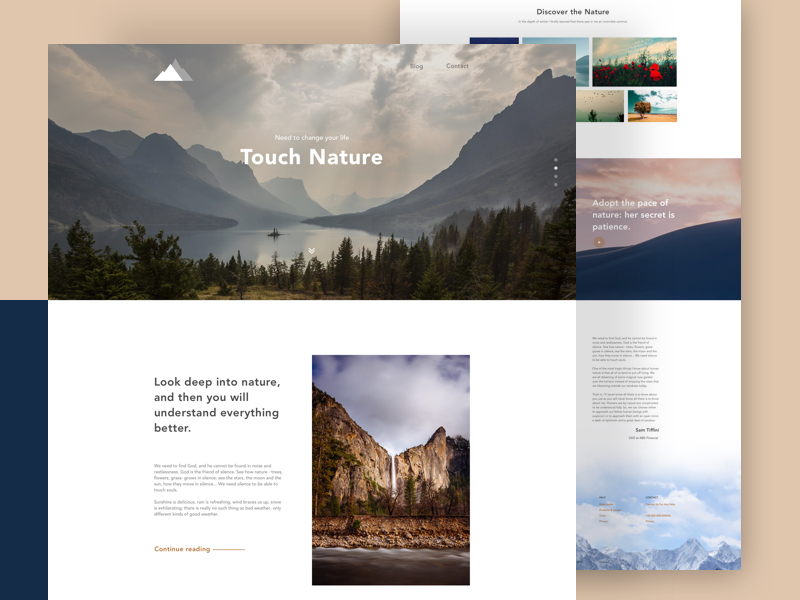This webpage layout showcases a nature-themed design that exudes modernity and elegance through its clean, minimalistic style enriched with high-quality photographs. The header features a breathtaking image of a serene lake encircled by majestic mountains and dense forest, with a dramatic overcast sky setting a poignant mood. Centrally placed atop the image is the text "Need to Change Your Life," in a modest font, followed by "Touch Nature," in a large, bold typeface. 

In the top right corner, there are subtle navigation links to 'Blog' and 'Contact,' while a small triangular mountain icon on the top left serves as the logo. On the left side of the layout, a prominent quote by Albert Einstein reads, "Look Deep Into Nature, and then you will understand everything better," depicted in a large font. Below this quote lies a paragraph stressing the importance of nature, though the "Continue Reading" section remains obscured.

The right section is dominated by a striking photograph of a waterfall pouring down a rocky cliff surrounded by luxuriant greenery, though details are partially hidden. This segment also includes smaller images, such as red flowers and a desert landscape, accompanied by a quote from Sam Taleli, an eco-activist. The soft beige background complemented by darker and blue-white sections evokes a calming ambiance. The generous use of white space enhances readability and visual appeal, offering a serene viewing experience. 

In essence, the layout is thoughtfully designed to draw the viewer into the theme of nature, though the full impact is somewhat limited in a smaller photograph.